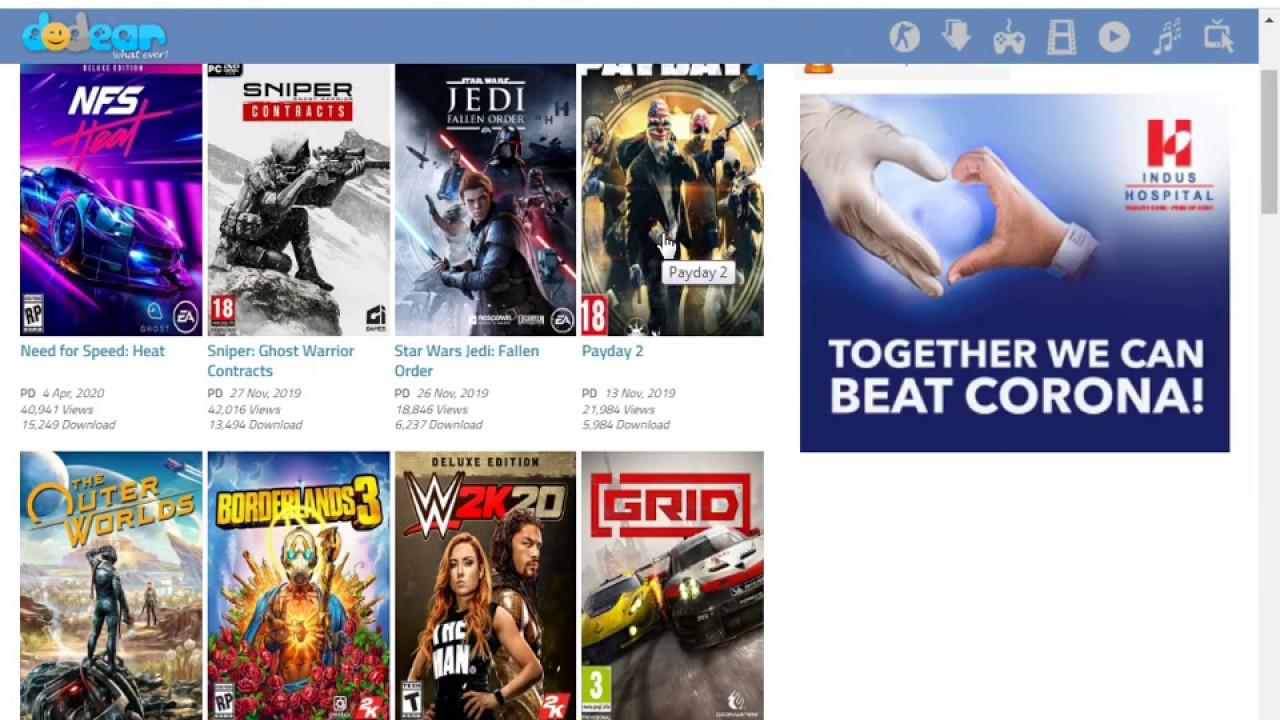On a light blue-gray background, the website "DODEAR" features prominently. To the right, there's a vertical bar containing circular icons representing various media forms, including a 'K,' a downward arrow, a game controller, a piece of film, a play button, a music note, and a TV. Below the icons are four video thumbnails arranged in a single line.

On the right side of the layout, a heart shape is created by two hands beneath the text "Together we can beat Corona," with the label "Indus Hospital" below it. 

The video thumbnails on the top row showcase the following titles:
1. "Need for Speed Heat"
2. "Sniper: Ghost Warrior Contracts"
3. "Star Wars Jedi: Fallen Order"
4. "Payday 2."

In the second row, only the titles are visible, which include:
- "The Outer Worlds"
- "Borderlands 3"
- "W2K20"
- "Grid."

The color scheme within the elements of the site includes a mix of purple, pink, gray, red, black, white, blue, green, yellow, and orange hues.